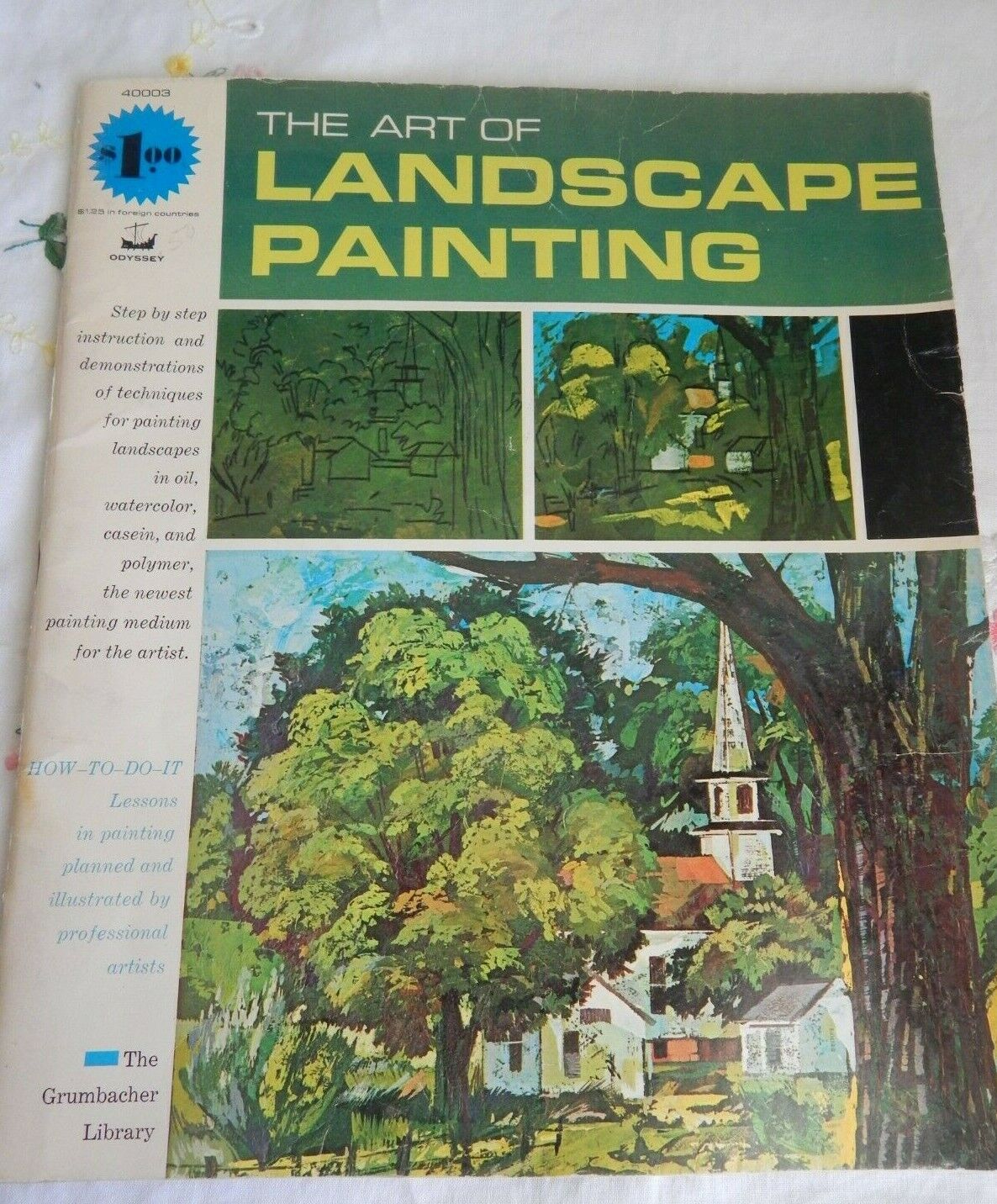This image showcases a book titled "The Art of Landscape Painting," prominently displayed on a clean, white surface. The cover of the book features a green background with the title text in contrasting colors: "The Art of" appears in small white letters at the top, while "LANDSCAPE PAINTING" is boldly printed in large yellow letters beneath it. 

Below the main title, the cover is divided into three blocks. The first block is filled with vibrant greenery, depicting green leaves drawn in various shades. The second block illustrates a variety of outdoor elements, such as plants and trees, contributing to the landscape theme. The third block, noticeably smaller, is empty and rendered in black.

The bottom section of the cover displays a completed landscape painting with a detailed scene: a white church with a steeple, a large green tree, assorted bushes, and additional trees extending towards the spine of the book. 

Additional text on the spine reads, “Step-by-step instructions and demonstrations of techniques for painting landscapes in oil, watercolor, casein, and polymer, the newest painting medium for artists.” This instructional guide, part of the Grumbacher Library, is priced at $1.99, marked by a blue price tag near the side edge of the cover. 

The overall design suggests that the book offers comprehensive, professionally illustrated lessons geared towards both novice and experienced artists looking to improve their landscape painting skills.